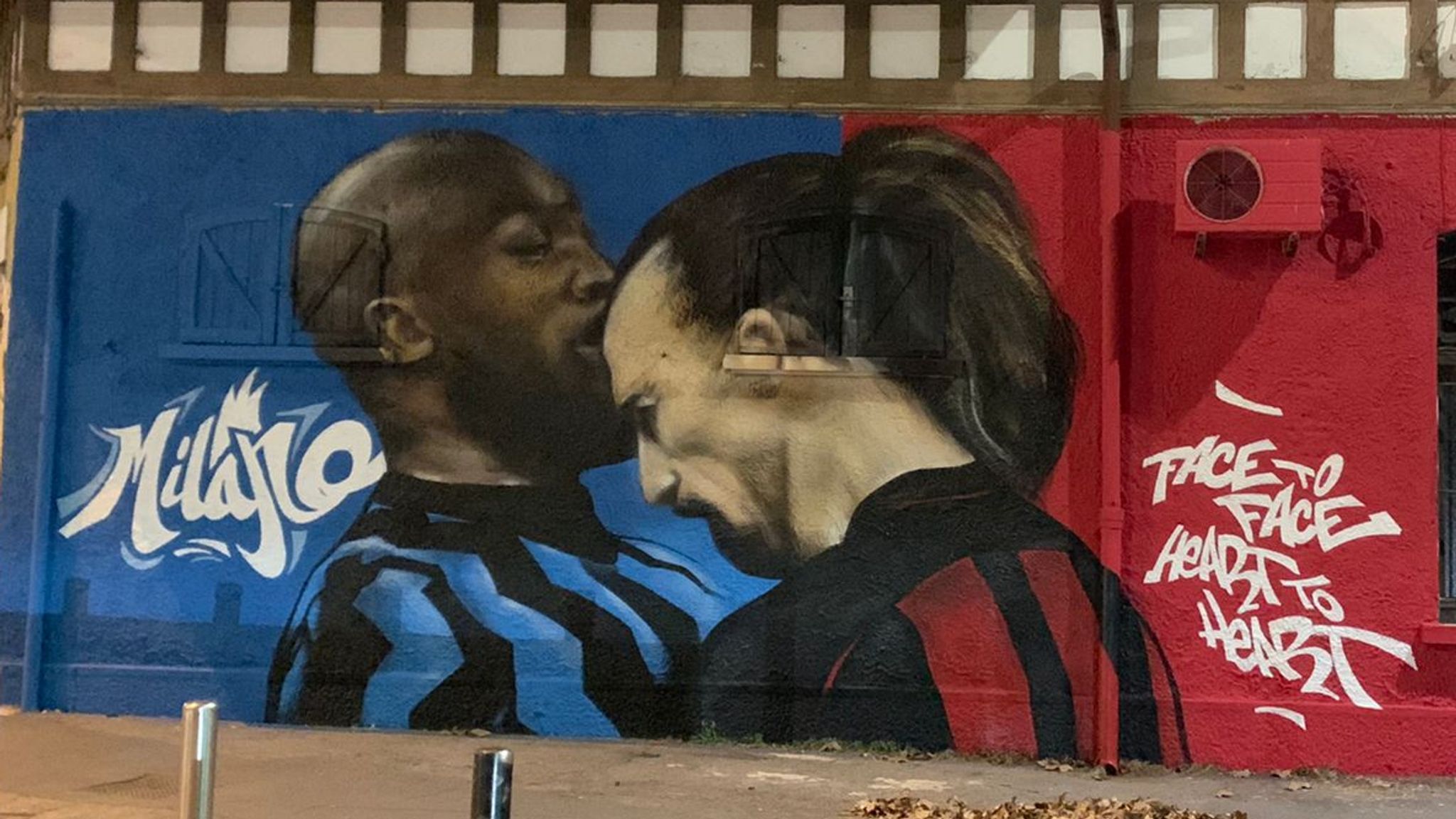The image is a photograph of a large, detailed mural painted on the side of a building, covering elements like shuttered windows and a cooling unit. The mural depicts two men in sports uniforms from opposing soccer (football) teams, embracing, with one man kissing the other on the forehead. The man on the left, with dark skin and wearing blue and black stripes, stands against a blue background. The man on the right, who appears to have lighter skin and his hair pulled back, is wearing red and black stripes and stands against a red background. Above the men on the left side, in white writing, are the letters "M-I-L-A-N-O," while on the right side, the phrase "face to face, heart to heart," appears in graffiti-style script. The men's expressions are fairly neutral, and at the bottom of the photo, you can see the sidewalk. This mural represents a poignant, harmonious moment between two athletes from rival teams, set in bold, contrasting colors.